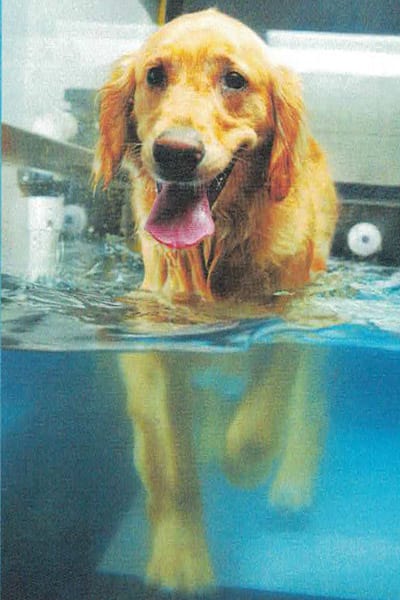This image features a golden retriever swimming in a pool with remarkably clear, blue water. The dog is oriented directly toward the viewer, its tongue cheerfully sticking out, contributing to an overall happy expression. Both the lower and upper halves of the image showcase the retriever: the lower half displays its legs paddling through the water, while the upper half shows its wet body above the waterline. The background transitions from lighter to darker blue hues as it reaches the waterline, with the pool's outer edges characterized by an off-white color and some black detailing. Additionally, the top part of the image includes white and black elements, possibly part of the pool's structure. The dog's characteristic golden fur and floppy ears are prominent, adding to the detail and vivacity of the scene.